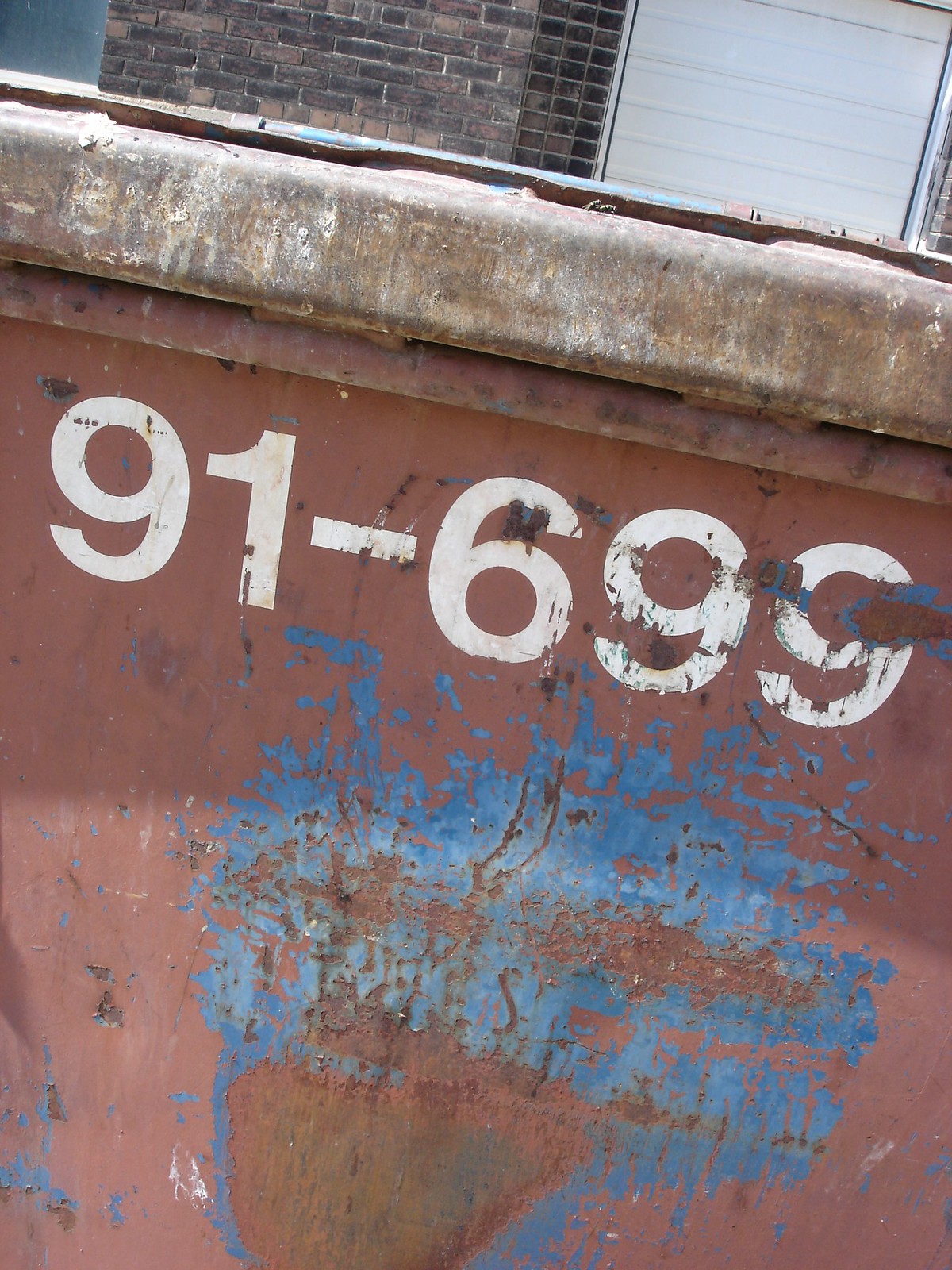The image shows a close-up of the side of a dumpster, originally painted a rusty red but now heavily weathered with chipped paint revealing patches of blue, brown, and rust. Across the top rim, which appears to have been white but is now dirty and rusted, are white block letters displaying the numbers "91-699," though some parts are chipped away. In the background, there is a multi-colored brick wall featuring varying shades of brown, beige, red, and even some almost black bricks, alongside a white garage door. The scene is set outdoors and the photograph is taken at a slight angle, making the left side appear higher than the right.